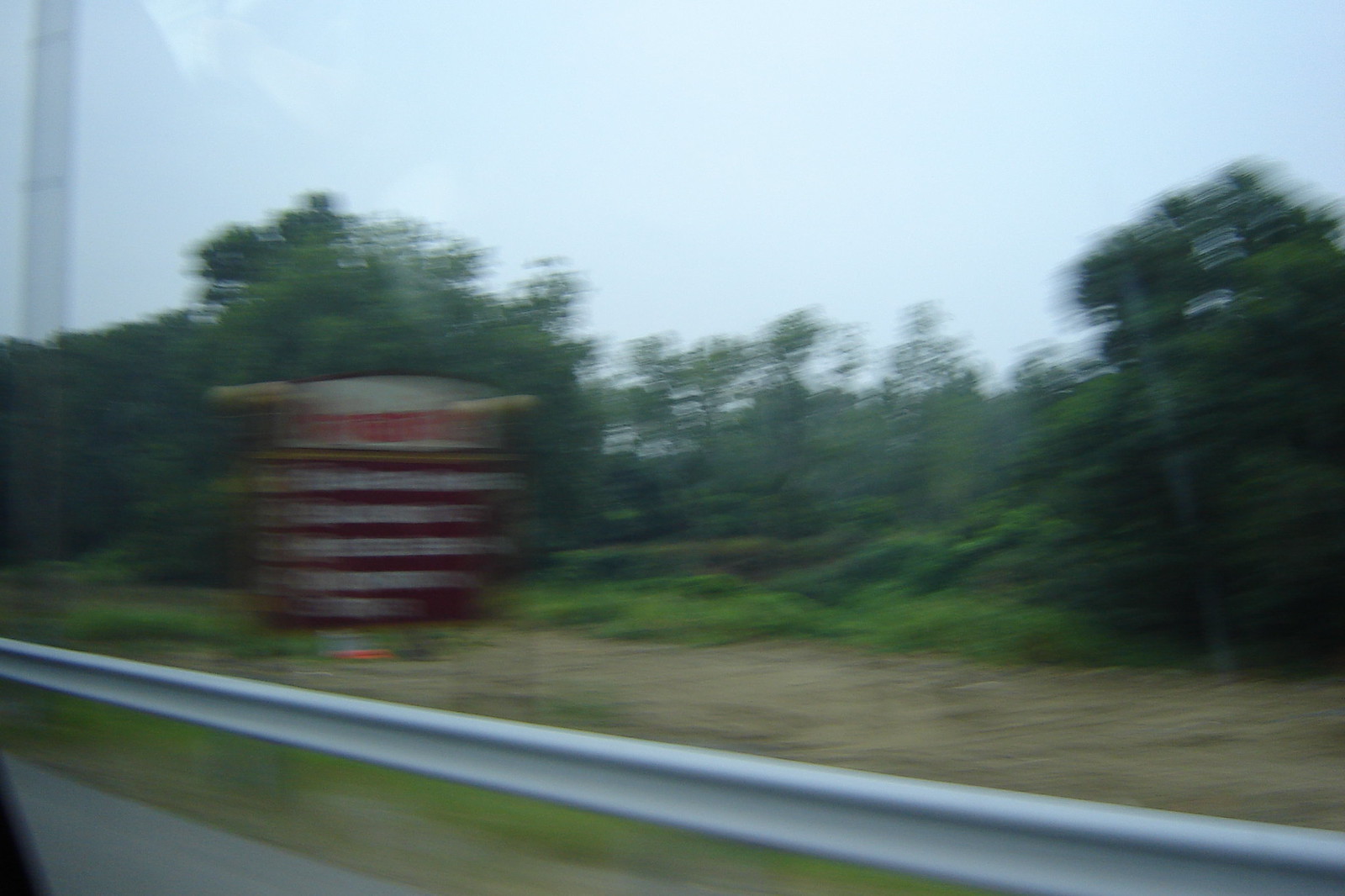This is a very blurry color photograph taken out of a moving car window, capturing a side view of a road scene. In the bottom left, part of the car window frame is visible with some asphalt next to it. Stretching diagonally from the bottom right to the upper left is a silver guardrail. The roadside area features a mix of dirt, greenery, and shrubbery, with a grassy field containing patches of dirt and sand. A brown and white sign stands along the forest edge, which is indistinct due to the blur; it has white text and a white section with red font at the top, flanked by yellow elements on either side. Beyond this, there's a densely wooded area with full, leafy trees under a blue sky. A faint reflection can be observed in the upper left of the image, and though no vehicles or people are present, the scene conveys the impression of speed and movement along a desolate stretch of road.